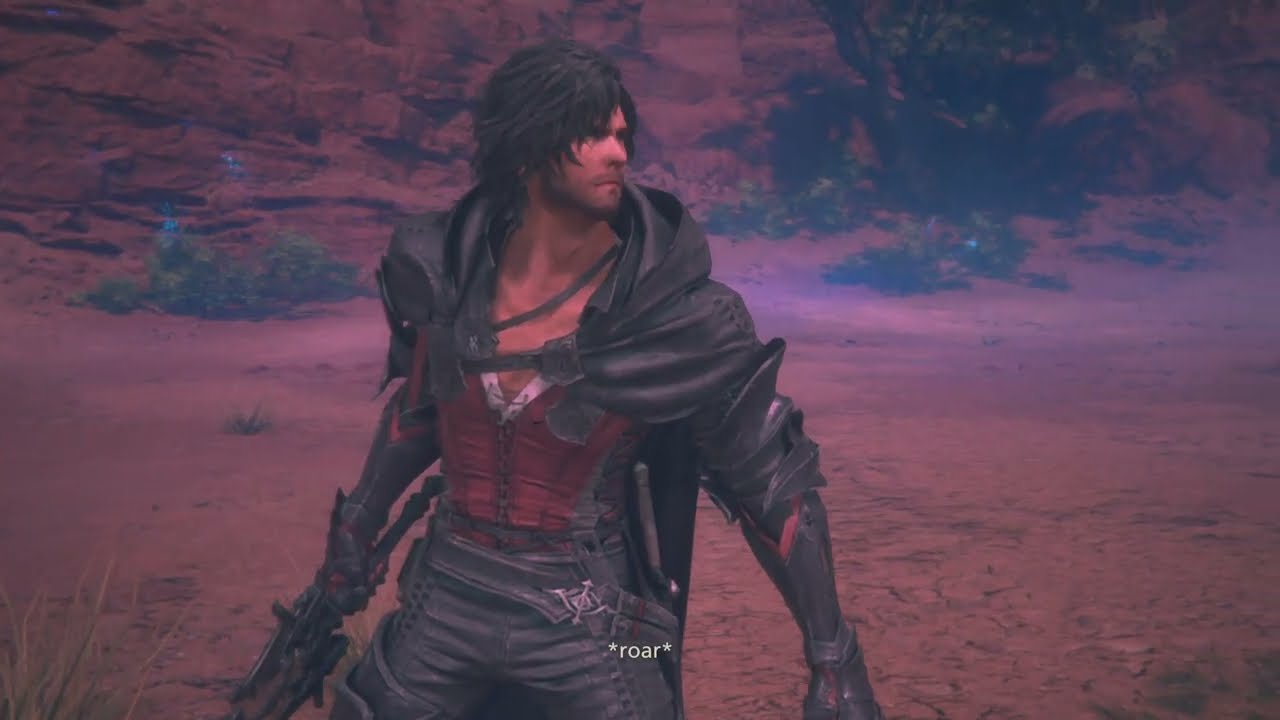In this image, we see a video game character set against a dry, arid backdrop, possibly during a cutscene. The character, a white male with fair skin and spiky black hair, is dressed in a detailed black leather outfit. He wears a black cloak, black leather pants with side stitching, and a red and white V-neck shirt tied up in the center, exposing his chest slightly. Over his arms, he has black armor adorned with red stripes. The character is equipped with a black weapon, likely a sword, in his right hand, with hints of a brown-handled knife in his pocket. He stands slightly to the left of the image, looking off to the right with a serious expression. 

The background features a landscape of orange-red dirt and large, light reddish rocks, indicative of a desert environment. Green shrubs and bushes are scattered throughout, with some larger ones on the right-hand side. The sky above is a rich purple, adding a mystical element to the scene, and there is a noticeable haze or fog rolling in, giving the backdrop a hazy appearance. At the bottom center of the image, there is text that reads "Roar," solidifying the dramatic tone of the scene. The overall setting suggests it is a still from a video game, capturing a moment of heightened tension.